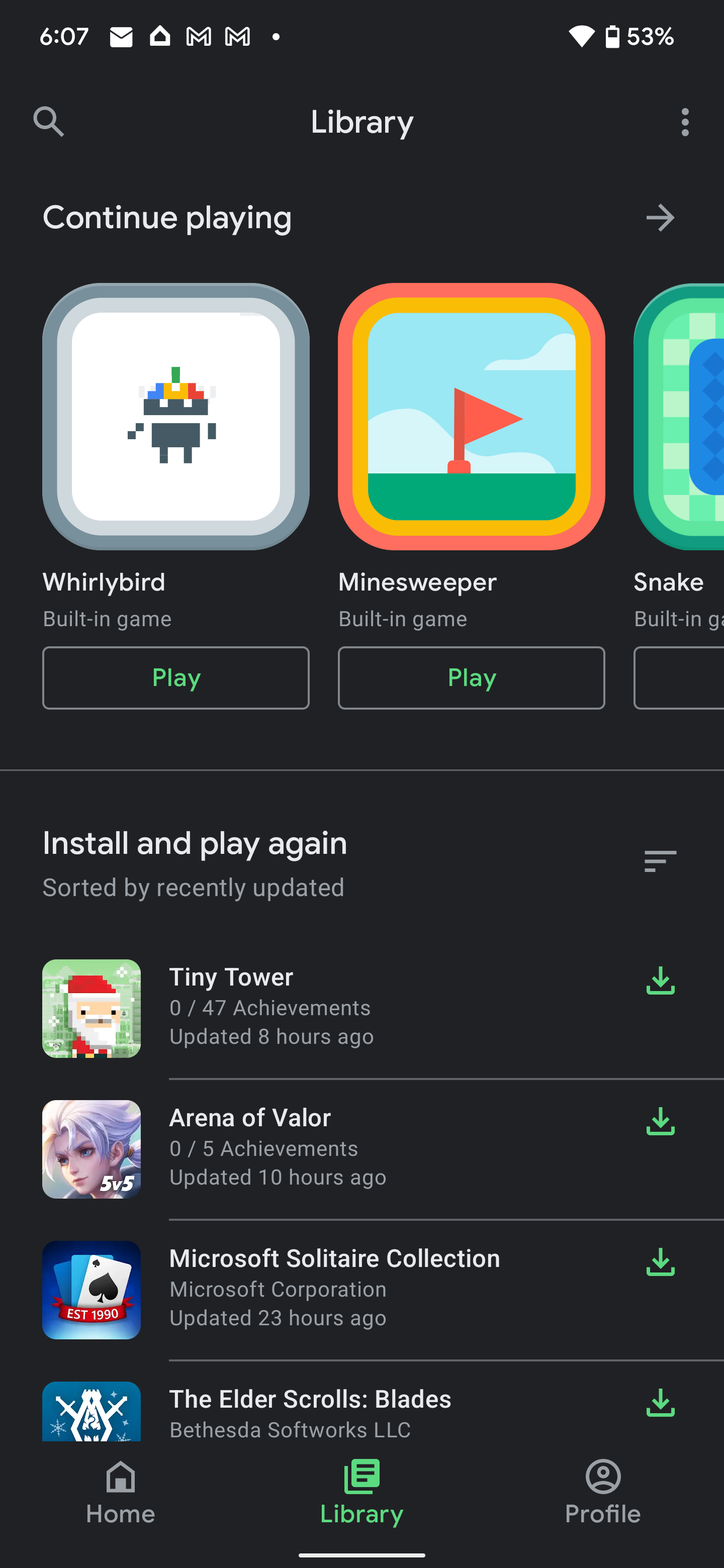This screenshot showcases the Google Play Store library section in dark mode. At the top lies the search bar labeled "Library," positioned centrally. Beneath this, on the left side, there's a section titled "Continue Playing." This section features three game icons, each accompanied by a play button underneath. The first icon represents the game "Bird," a built-in game, followed by "Minesweeper," another built-in game.

The next section is labeled "Installed and Play Again," sorted by recently updated games. This portion contains four game icons:
1. "Tiny Tower," updated 8 hours ago, depicted with a Santa Claus figure in 2D pixel art.
2. "Arena of Valor," updated 10 hours ago, showcasing an anonymous character with lilac hair.
3. "Microsoft Solitaire Collection," updated 23 hours ago, illustrated by a spade card.
4. "The Elder Scrolls: Blades," represented by a shield flanked with two swords.

To the far right of each row in this section, there is a green download icon for quick access.

At the footer of the image, there are three primary icons: a home icon, a library icon (highlighted in green), and a profile icon, indicating the user's current navigation path.